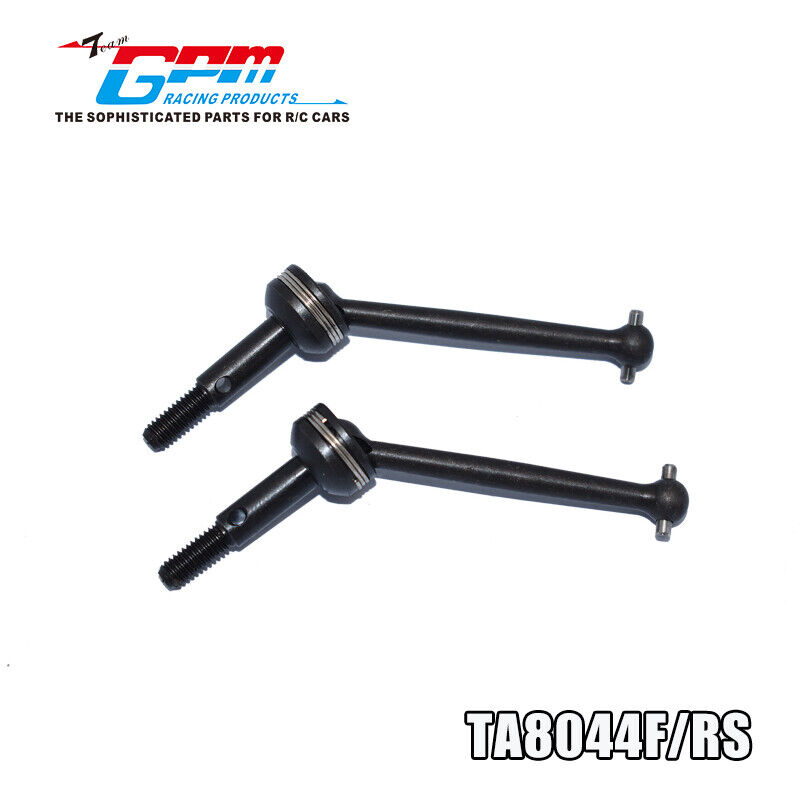The image features two identical, sophisticated black metal stabilizer bars designed for RC cars, likely manufactured by GPM Racing Products. The top corner of the image displays the GPM logo in half red and half blue letters, followed by "Racing Products" in blue letters with a small arrow and "The sophisticated parts for RC cars" in small black letters. The bars, labeled with the part number "TA8044F/RS" in large black block letters outlined in white at the bottom of the image, are almost L-shaped or V-shaped, with a round part connecting the two sections. Each stabilizer bar has a threaded end with grooves for screwing into another component. The other end features a rod and swivel mechanism with knobs protruding from the sides, indicating their role in providing stability and maneuverability to the RC vehicles. The image itself has no background color or border.